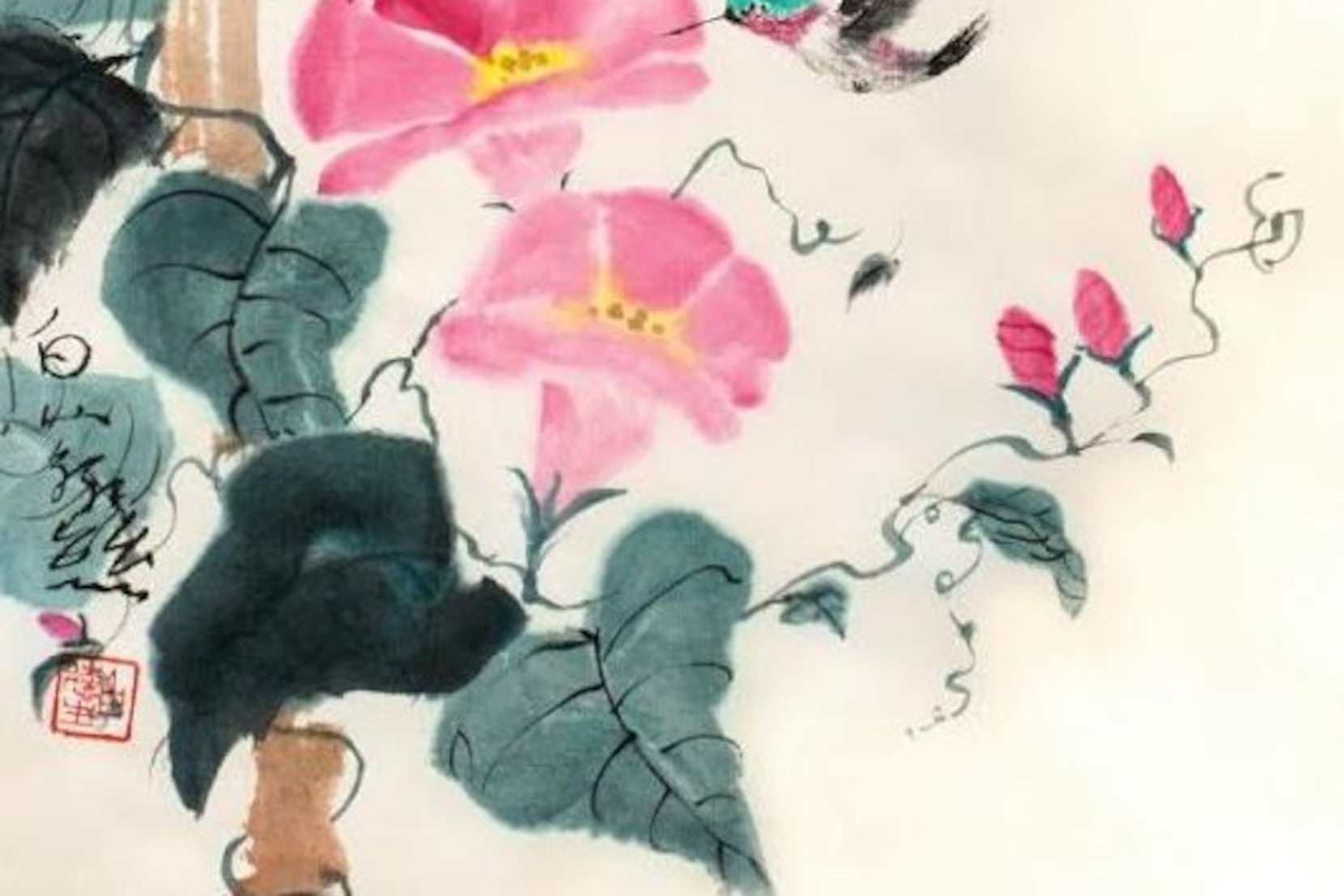This is a detailed watercolor painting with a light beige background, featuring prominent Asian influences, likely Japanese. On the left-hand side, there is intricate handwritten or brushed Japanese calligraphy, complemented by a small red stamp containing additional Asian characters, presumed to be the artist's signature.

The main subject of the painting is a remarkably graceful vine, which starts from the bottom left corner, extends diagonally upwards, and curves elegantly towards the right side. The vine is adorned with lush, dark green and pale emerald heart-shaped leaves scattered along its thin, winding stem. Interspersed among the leaves are delicate pink flowers, each with distinctive petals that form a vibrant circle around a bright yellow center. 

Three unopened buds at the vine's end hint at the life waiting to bloom. A gentle brown stem supports the entire vine structure, adding to the painting’s earthy feel. Adding a touch of dynamism, a beautifully detailed hummingbird is depicted feeding on one of the flower centers. The bird showcases a teal head, a red throat, a white belly, and black wings, all captured with the fluidity typical of watercolor art. The painting's soft lines and blend of colors create a sense of tranquil natural harmony.